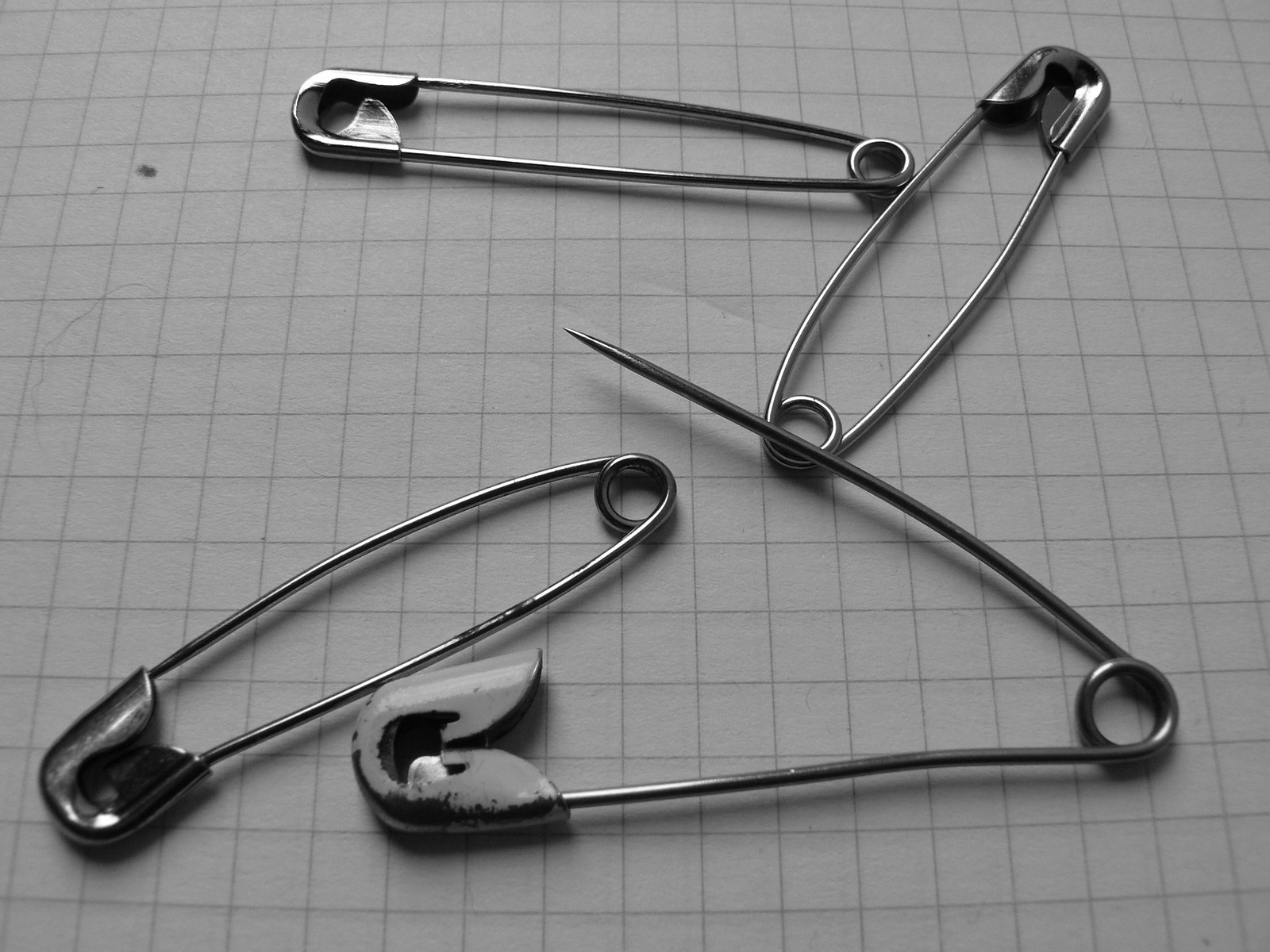This image features a close-up photograph of four well-used safety pins arranged on a piece of faintly lined graph paper. The background reveals subtle details such as a stray hair and a small dark smudge on the left-hand side, probably from a pencil. Among the pins, three are fully closed, while the bottom right pin stands out as the largest and only open one, revealing its sharp needle-like point. This open pin shows significant wear, with its once white paint chipped away, exposing the underlying black or tarnished silver metal. The bottom left pin appears slightly bent and scuffed where its pin meets the latch, highlighting its frequent use. The safety pins, all made of steel, display a variety of weathering effects, especially the dull gray patches from the chipped paint. Their arrangement on the grid paper is somewhat triangular, with the top and left three pins placed diagonally from the bottom left to the top right, and the top left pin spanning horizontally.